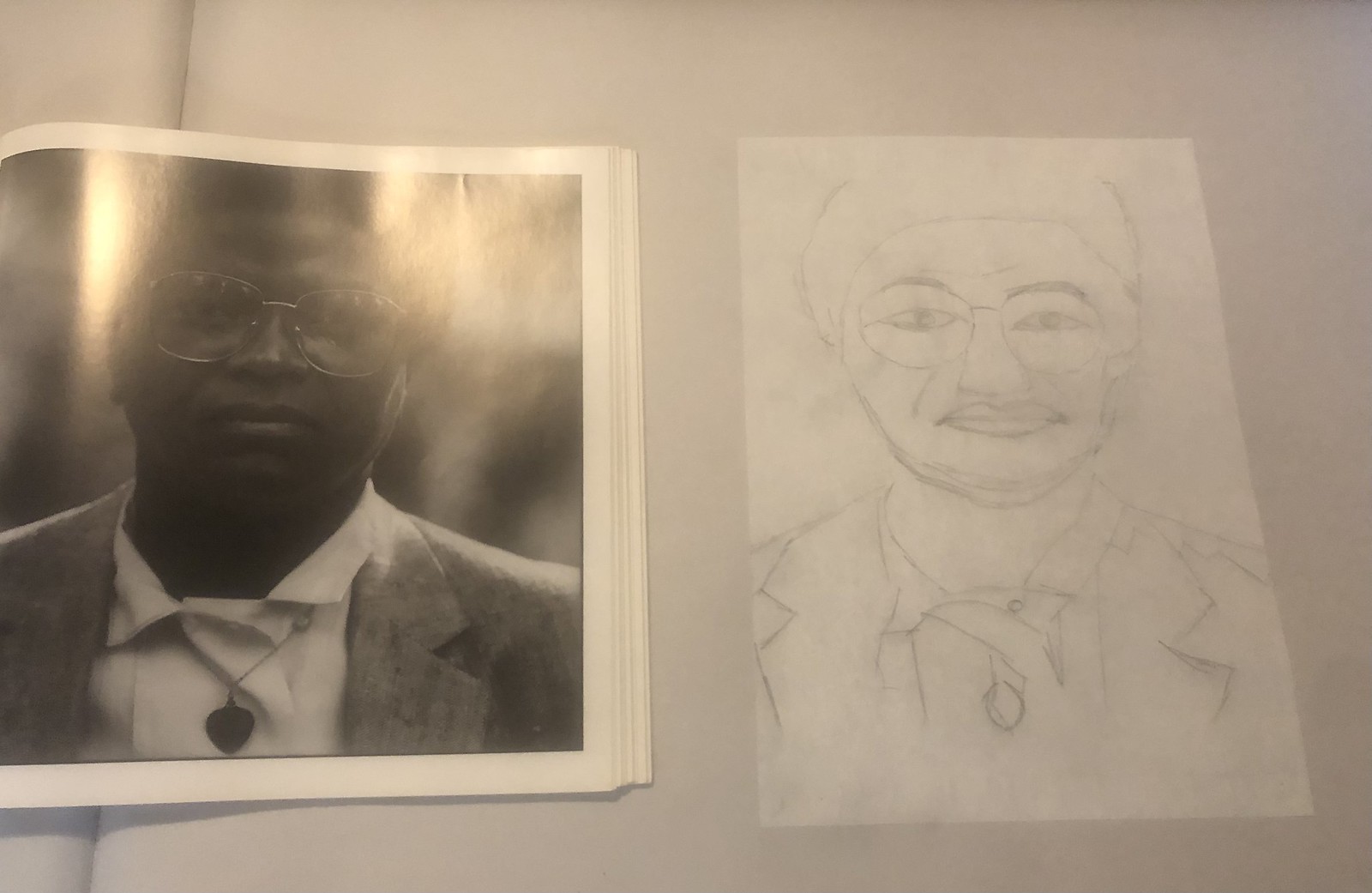The image features a black and white photograph of an African-American man on the left, wearing large glasses, a white shirt with a collar, a suit jacket, and a pendant resembling a Saint Christopher necklace. The glossy nature of the photograph is apparent, with light reflecting off the surface creating striking yellow streaks. The man appears serious in expression. To the right of the photograph, there's a pencil sketch of the same man on a piece of paper, capturing his likeness reasonably well despite some imperfections. The background is predominantly gray, with light and shadows creating various shades of gray. The image composition follows a left-to-right rectangle format with a subtle line dividing the darker left side from the lighter right side, enhancing the multi-faceted visual effect.